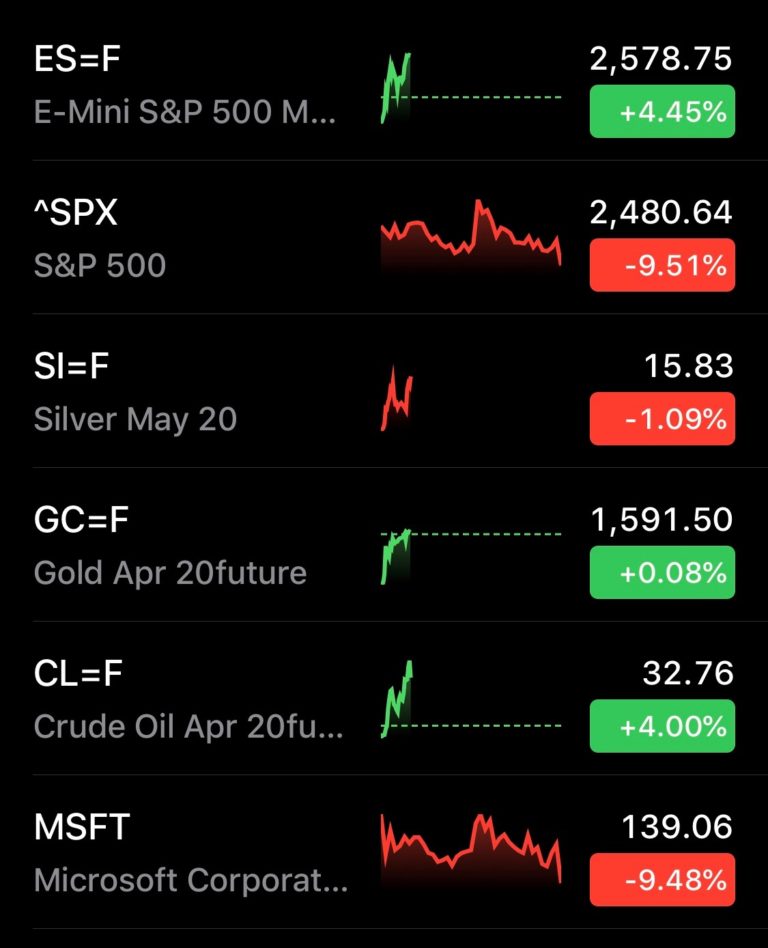The image features a dark black background with gold highlights, creating an elegant contrast. It appears to show a detailed list of financial assets and their respective performance metrics, organized in a two-column layout.

On the left side of the image, there are six items listed with information extending to the right:

1. **ES=F**: 
   - **Expanded text**: E-mini S&P 500
   - **Value**: 22,578.75 
   - **Change**: +4.45%
   
2. **SPX**: 
   - **Expanded text**: S&P 500
   - **Value**: 2,480.64 
   - **Change**: -9.5%
   
3. **SI=F**: 
   - **Expanded text**: Silver May 20
   - **Value**: 15.83 
   - **Change**: -1.09%
   
4. **GC=F**: 
   - **Expanded text**: Gold April 20 Future
   - **Value**: 1,591.50 
   - **Change**: +0.08%
   
5. **CL=F**: 
   - **Expanded text**: Crude Oil April 20 Future
   - **Value**: 32.76 
   - **Change**: +4.0%
   
6. **MSFT**: 
   - **Expanded text**: Microsoft Corporation
   - **Value**: 139.06 
   - **Change**: -9.48%

The text colors used in the image include white for most text, gray for secondary information, green to indicate positive changes, and red to denote negative changes, all set against a sophisticated black background. The contrast between the colors and the dark backdrop ensures clear readability while emphasizing the financial data's fluctuations.